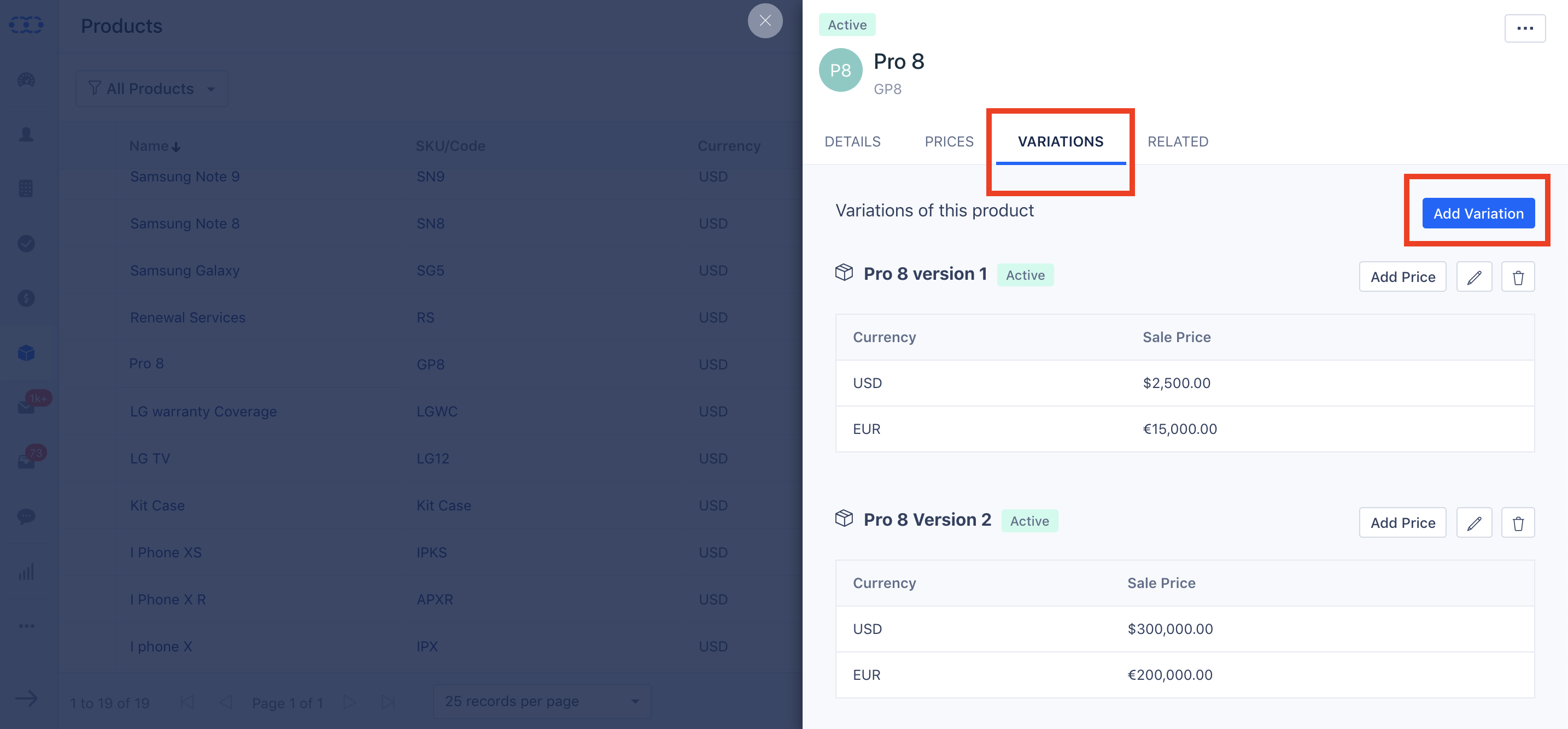A detailed and cleaned-up descriptive caption for the provided image could be:

"A screenshot from a device displays a partially obscured interface for managing product listings. The left side of the screen is predominantly blacked out, with faint, grayed-out text that includes product names such as Samsung Galaxy Note, Samsung Note 8, and Samsung Note 9, along with various columns comprising product details. In contrast, the right side of the screen is clear and features a white background. At the top, the word 'Active' is highlighted in a gray box, followed by the listing 'Pro 8' next to a green circle labeled 'P8'. Below, there's a sectioned layout for 'Details', 'Prices', 'Variations', and 'Related'. Notably, the 'Variations' section is marked with a red rectangle and underlined with a blue line. Within this section, there's a prompt stating 'Variations of this product', accompanied by a blue 'Add Variation' button, which is also highlighted with a red rectangular outline."